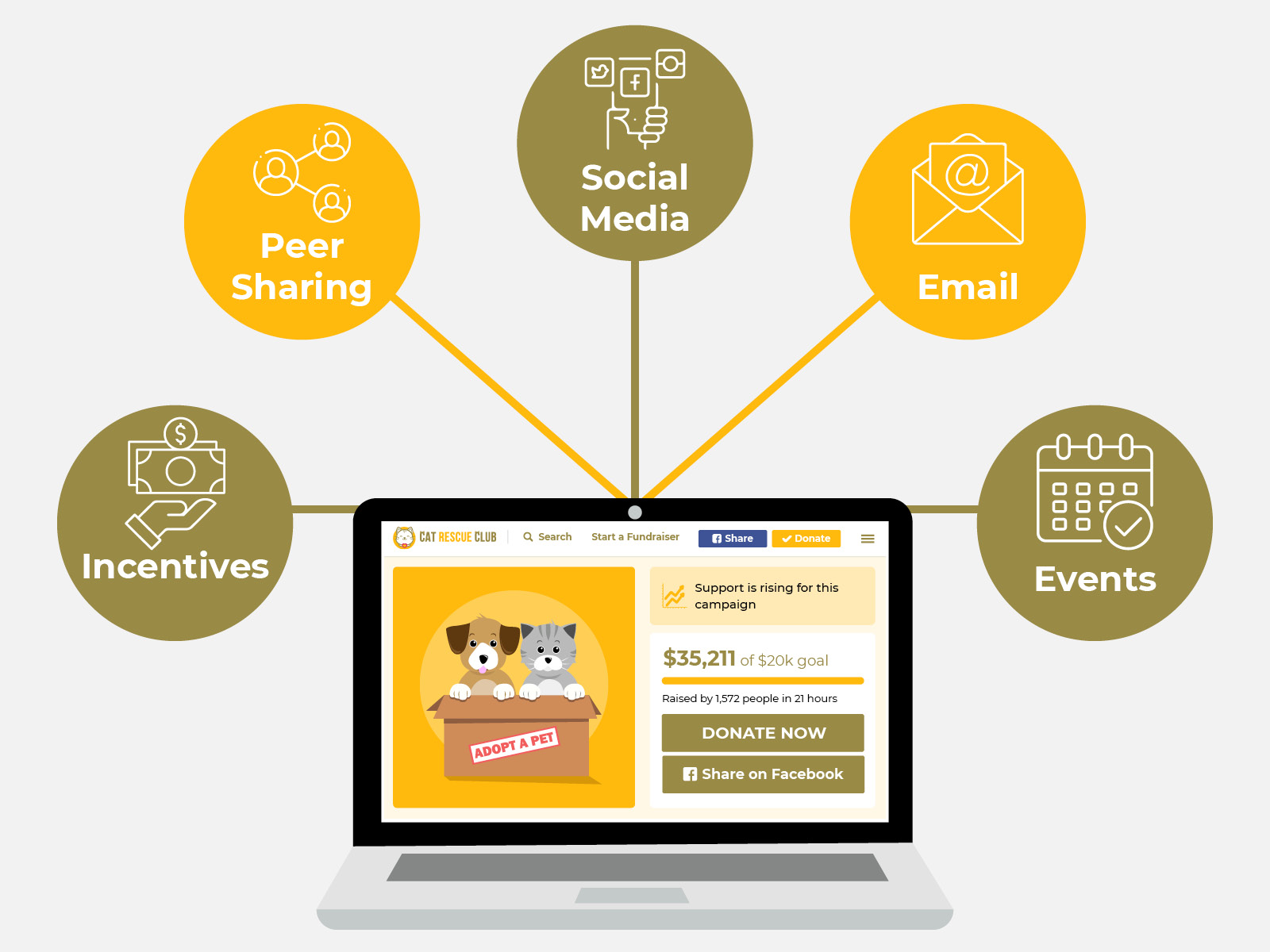This image is a detailed social media informational graphic illustrating a laptop screen featuring a fundraising website for the "Cat Rescue Club." The website's header in the upper left corner includes a "Cat Rescue Club" title accompanied by navigation options such as "search," "start a fundraiser," "share on social media," "donate," and a hamburger menu for additional options. The laptop, depicted with a gray and black design, showcases a central image of a dog and a cat in a box with the label "Adopt a Pet." To the right, the website displays a progress indicator stating "support is rising for this campaign" in an orange banner, followed by details of the funds raised: "$35,211 of a $20,000 goal, raised by 1,572 people in 21 hours." Below this, prominently placed buttons encourage viewers to "Donate Now" and "Share on Facebook." Surrounding the top of the laptop are five connected circles in alternating tan and yellow colors, each detailing various aspects of the campaign's strategy: "Incentives" with an icon of a hand holding money, "Peer Sharing" featuring head outlines, "Social Media" with a hand holding a phone displaying multiple emblems, "Email" indicated by a note card entering an envelope, and "Events" marked by a calendar with a check mark. The background is predominantly gray, emphasizing the visual elements of the fundraising effort for pet adoption.